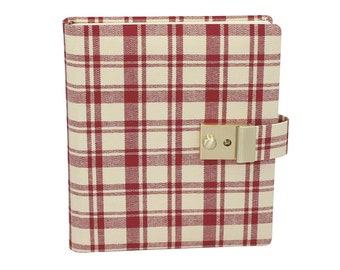The image depicts a vertically positioned cloth-covered diary resting on its long edge, set against a plain white background. The front cover features a sophisticated dark red and cream plaid pattern, reminiscent of designer styles such as Ralph Lauren or polo patterns. The plaid incorporates vertical and horizontal stripes, creating an upscale aesthetic. The diary is secured with a belt that has a silver clip, seemingly incorporating a magnetic fastening system that can be released by pressing a button on the belt. The clasp appears to have a small decorative element, possibly a pearl-like feature, and might be attached with a tiny screw. Although the image offers a view of the front, top, and side of the diary, the back isn't visible, nor can the internal pages be examined to determine if they are lined or unlined. The pages that are visible, however, are cream-colored, matching the cover's hue.